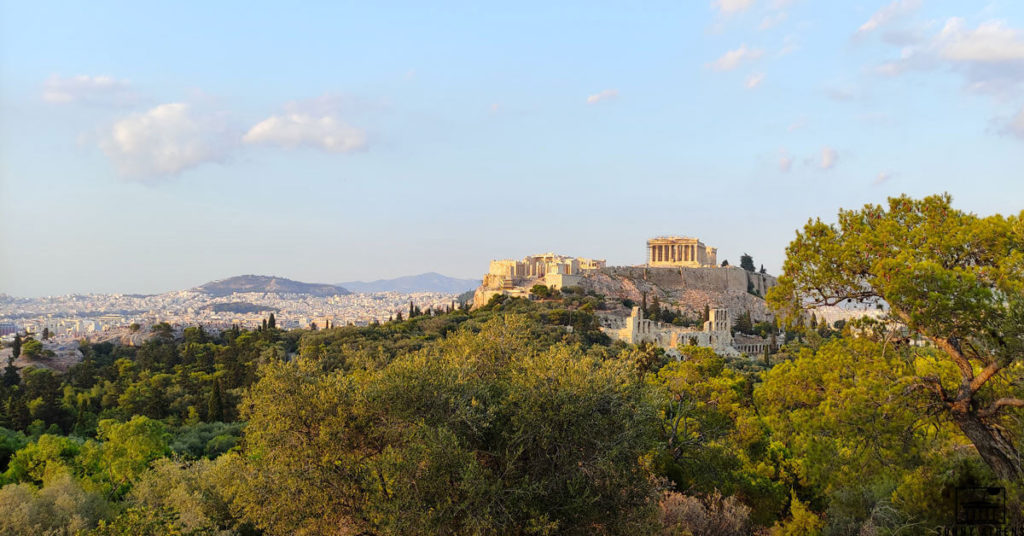The outdoor, daytime photograph showcases a stunning, expansive view of the ancient Parthenon in Athens, nestled atop a rocky cliff. This iconic structure, characterized by its imposing vertical columns and triangular roof, occupies the middle right section of the image, overlooking a vast cityscape. Surrounding the Parthenon, a dense concentration of green trees extends in the foreground with lighter shades closer to the viewer, transitioning to darker hues further back. At the base of the cliff are additional marble ruins, including pillars and fragmented walls, hinting at the historical depth of the site.

The left half of the photo reveals a sprawling modern city with countless white buildings seamlessly blending into each other, set against a backdrop of modest hills and mountains. The sky above is a serene light blue, adorned sparsely with white clouds mostly congregated to the left and top right corners of the image. The composition captures the harmonious juxtaposition of ancient and modern elements within the landscape, illustrating a timeless connection between the past and present.